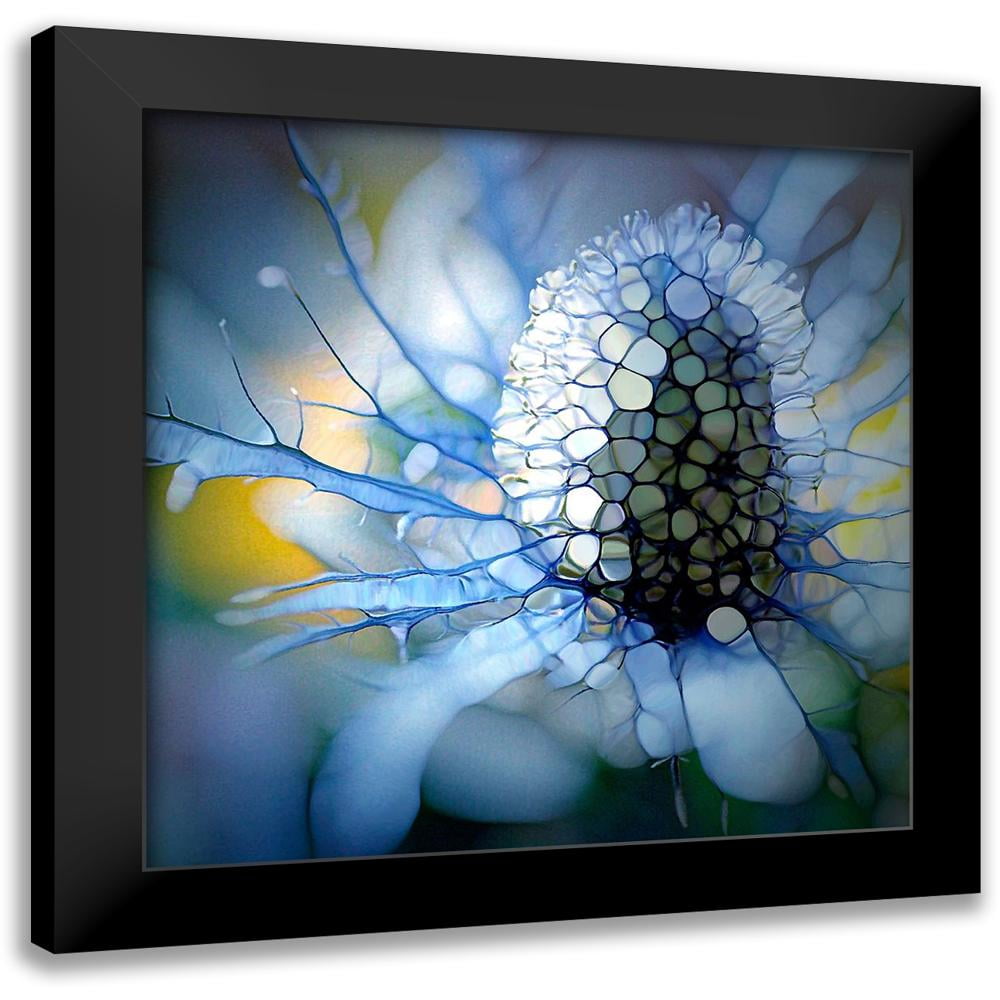This product listing photograph showcases a framed digital rendering of a floral pattern, encapsulated in a sleek black rectangular frame against a plain white backdrop. The artwork within the frame appears to be an extreme close-up of a flower, depicted in a style reminiscent of stained glass or broken glass. The central part of the flower is composed of numerous small white pieces, with blue and green petals radiating outward. These elements are intricately detailed, creating a mosaic-like texture that lends a surreal and almost mystical quality to the image. The photo also includes hints of yellow, further adding to the color complexity. The overall palette is primarily cool, featuring dominating shades of white, blue, and green, while background details remain blurry, emphasizing the flower’s elaborate design.